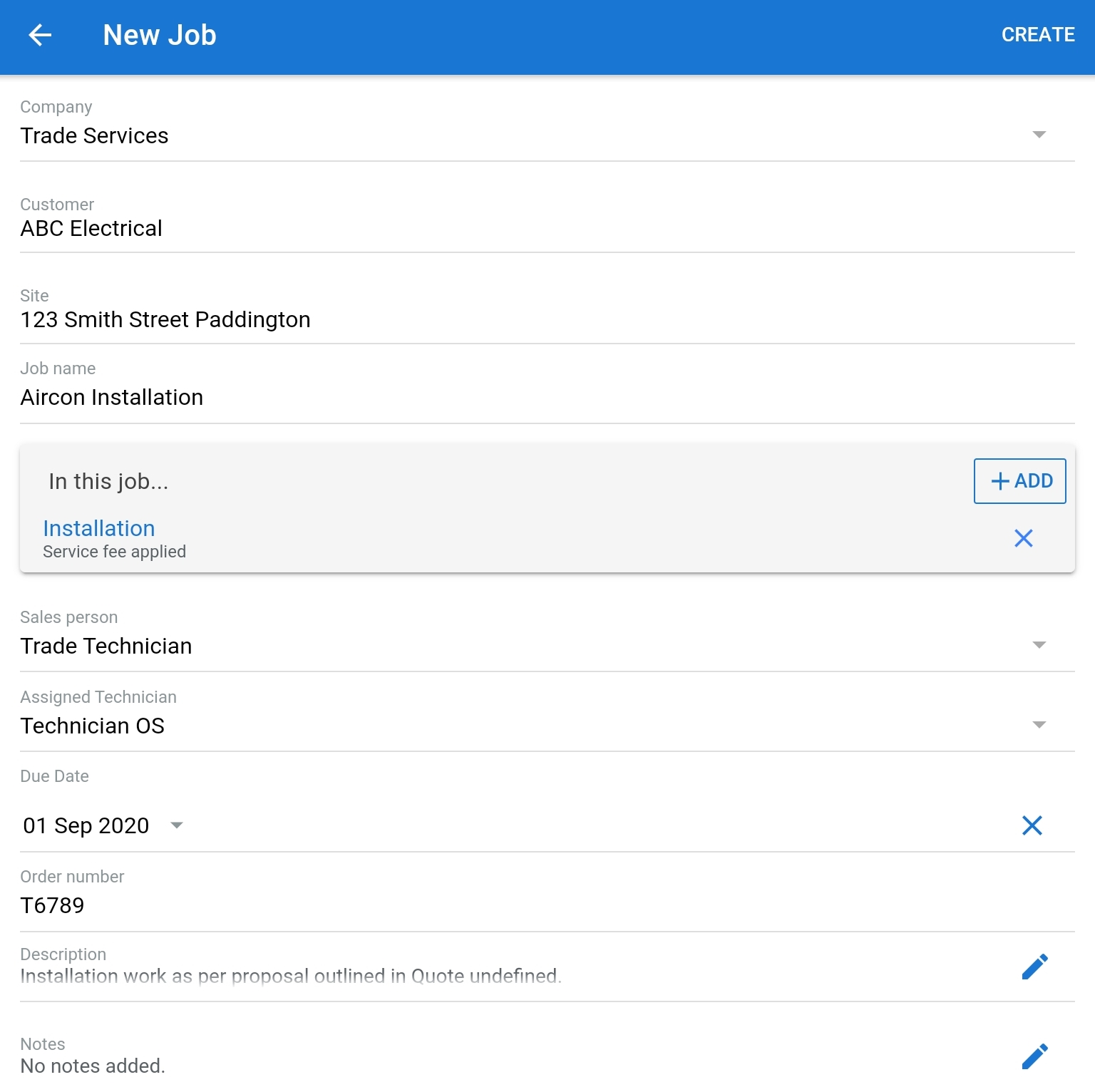The image features a user interface for a job management system. At the top, there is a blue strip with a left-angled arrow labeled "New Job" on the left and a "Create" button on the right. Below this strip, the background is predominantly white. The text "Company Trade Services" is displayed with a dropdown menu on the right side.

A series of gray divider lines organize the following information:
1. "Customer: ABC Electrical"
2. "Site: 123 Smith Street, Paddington"
3. "Job Name: Air Con Installer"

Beneath these details, there is a horizontally elongated rectangle. On the left side of this rectangle, the text reads "In this job... Installation Service Fee Applied," and on the right side, there is a blue "+" (Add) button next to a blue "X" (Delete) button.

Further down, the interface lists various fields, each separated by lines:
- "Salesperson"
- "Technical Trade Technician"
- "Assigned Technician"
- "Technician OS"
- "Due Date: 017/2020"
- "Order Number: T6789"
- "Description: Installation work as proposed in Quote (undefined)."

Additionally, there is an "X" mark next to the due date, and dropdown menus for both the Trade Technician and Trade OS fields. The Description and Notes sections also include pencil icons on the right side for editing.